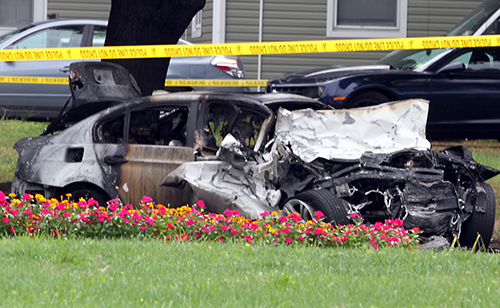The photograph depicts a harrowing scene of a devastating car crash, with a specific focus on a severely charred and crumpled vehicle that appears to have caught fire. The car, which may have originally been white or tan, is now blackened like charcoal, with the front end completely smashed and the interior utterly destroyed. The front hood is folded back onto the windshield, and the side door is demolished. The vehicle is surrounded by "police line, do not cross" tape, cordoning off the area. The scene is incongruously set against a backdrop of vibrant green grass and an array of bright, colorful flowers in the foreground, creating a stark juxtaposition of life and beauty against the tragedy. Beyond the police tape, several other cars are visible, and the location appears to be near a building with gray wet paneling and white stripes, possibly indicating a residential or park area. Overall, the image captures a poignant contrast between the vivid hues of the blooming flowers and the bleak remains of the incinerated car, illustrating the fragility of life amidst the devastation.